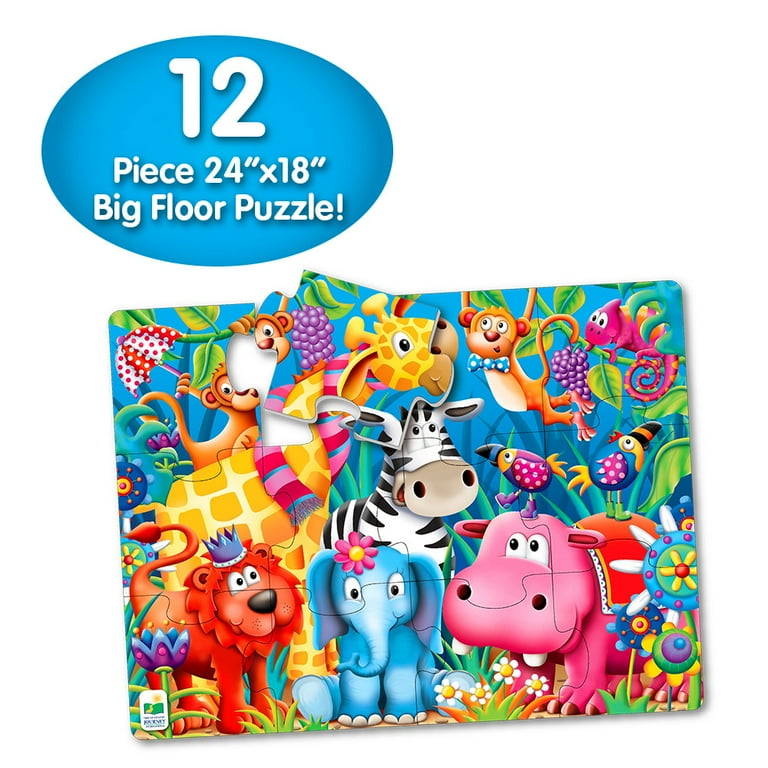The image is a lively advertisement for a colorful, 12-piece, 24-inch by 18-inch big floor puzzle designed for children. At the top of the image, a prominent blue oval bubble with white text highlights the puzzle's specifications: "12 piece, 24 inch by 18 inch, big floor puzzle." Directly below this text, the featured puzzle illustration showcases a vibrant, animated jungle scene set against a predominantly blue background. The scene is a whimsical menagerie of happy, smiling animals, including a red lion wearing a crown, a blue elephant adorned with a pink flower, a pink hippopotamus with dancing toucan birds on its back, a cartoonish zebra, a large giraffe, and several other birds and monkeys. The image cleverly reveals how the puzzle pieces fit together by having one of the top left pieces slightly removed, giving a glimpse of the nearly completed puzzle. The overall design is aimed at capturing the attention and imagination of young children.